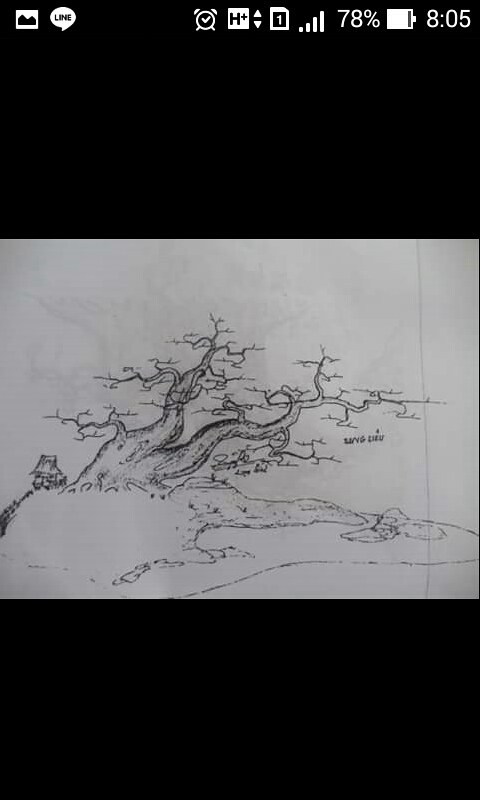This image is a screenshot captured from a mobile phone, divided into three distinct sections. The top 30% of the image features a black background adorned with various white icons typically found on a phone's status bar. Starting from the left, the icons include an image symbol, followed by the Line app icon resembling a chat bubble. After a space, the right side showcases several more icons: an alarm clock, a white square with a black H and plus sign, two overlapping triangles, an SD card symbol with a number one inside it, signal bars indicating four bars of signal strength, a battery icon showing 78% charge, and the time reading 8:05.

The middle section of the screenshot appears to be the main focus. It includes an image that seems to be either a photo or a screenshot of a hand-drawn illustration executed on white paper with black pen or pencil. The illustration itself is ambiguous, resembling either a leafless tree or a tree branch, potentially merging into a map-like form, showcasing intricate details.

The bottom part of the image is another black bar, balancing the composition and framing the central illustration effectively.